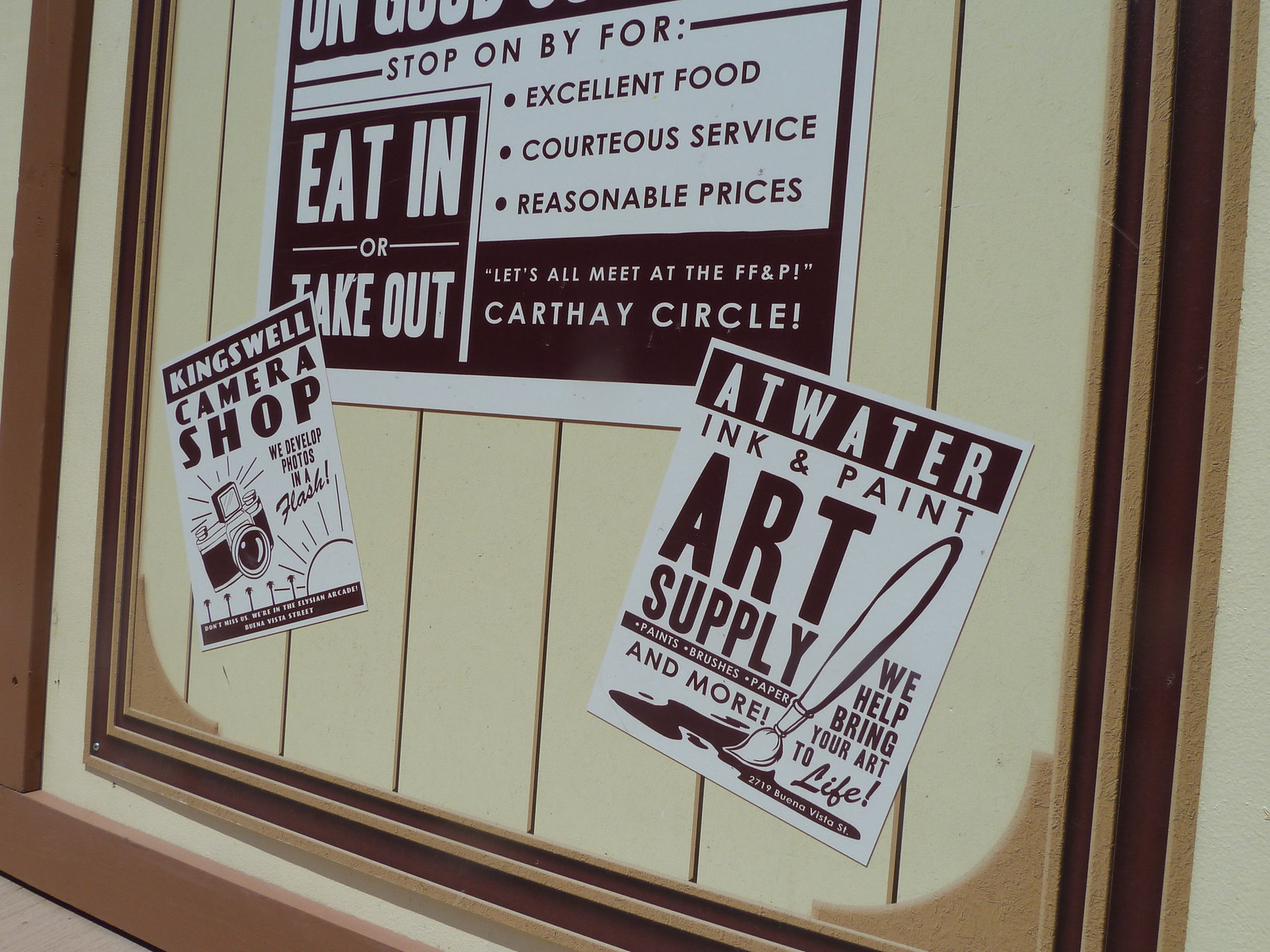In the image, you see the bottom half of a framed poster that showcases various black-and-white advertisements mounted on a series of vertical wooden slats. The frame is a light tan or brownish color. Centered at the top of the visible portion is a partially cropped, large black-and-white sign that reads, "Stop on by for excellent food, courteous service, reasonable prices. Let's all meet at the FF&P Carthay Circle. Eat in or take out." Directly beneath this, to the bottom left, is a slightly tilted poster for the Kingswell Camera Shop, featuring an illustration of a camera with a sun and the text, "We develop photos in a flash." On the bottom right, also tilted, is another ad for Atwater Ink and Paint Art Supply, including an image of a paintbrush painting black ink and the text, "Paints, brushes, paper, and more. We help bring your art to life," along with the partial address "2719 Buena Vista Street." The interior of the poster background is tan with dark maroon or almost black text and designs.